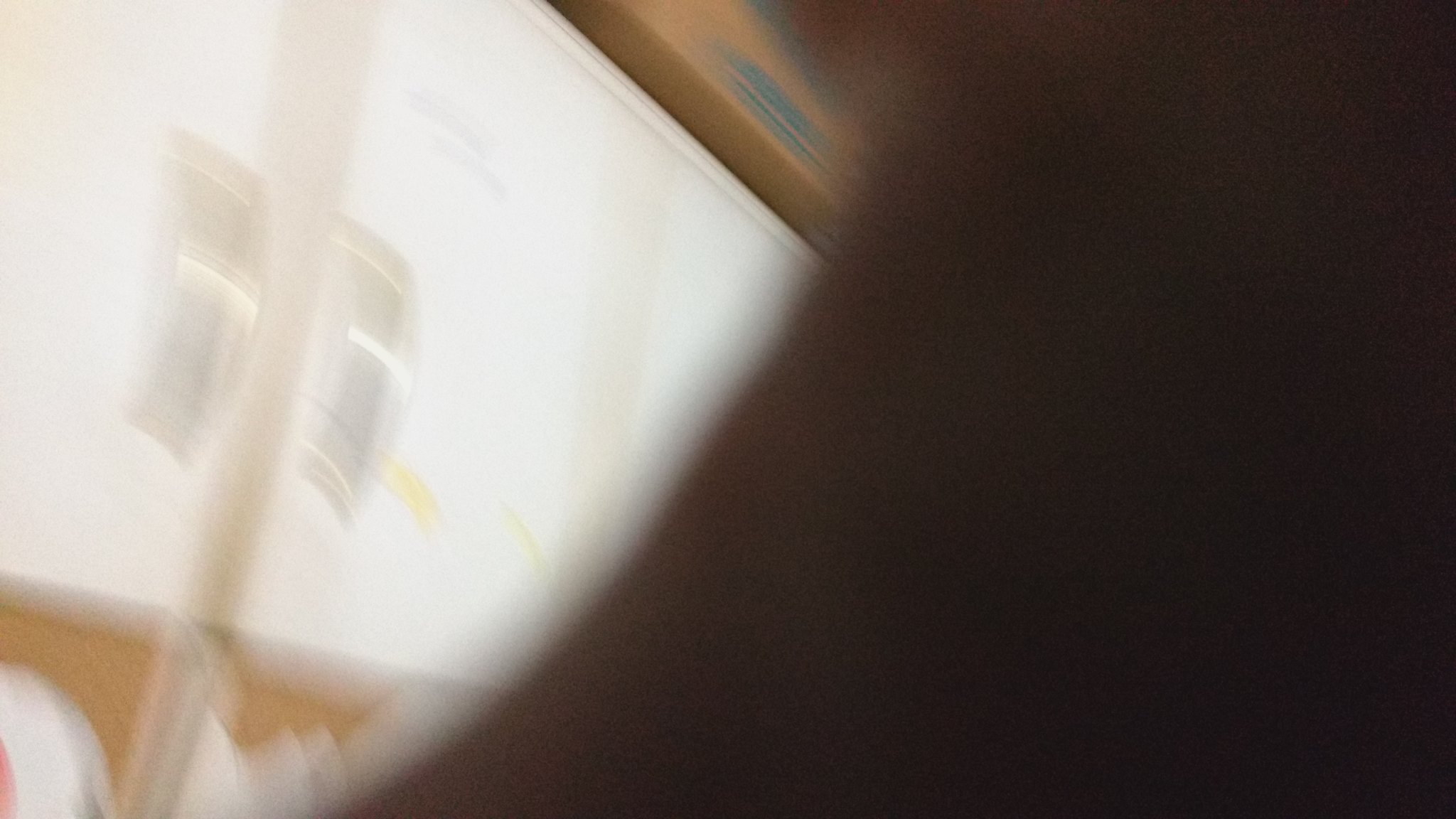This image is blurred and predominantly dark, particularly on the right side. The darkness suggests the presence of a silhouetted figure, possibly delineating a shoulder and part of a head. On the left, the image is lighter, featuring a white wall, albeit also blurred. A wooden panel runs along the top of this wall, possibly housing a vent. Additionally, an object resembling an IV stand, typical of a hospital setting, is visible. The background contains another wooden element that resembles a headboard, further hinting at a hospital environment. This scene might depict someone sitting beside another person, possibly in a hospital room, although this interpretation remains uncertain due to the vagueness and blurriness of the image.